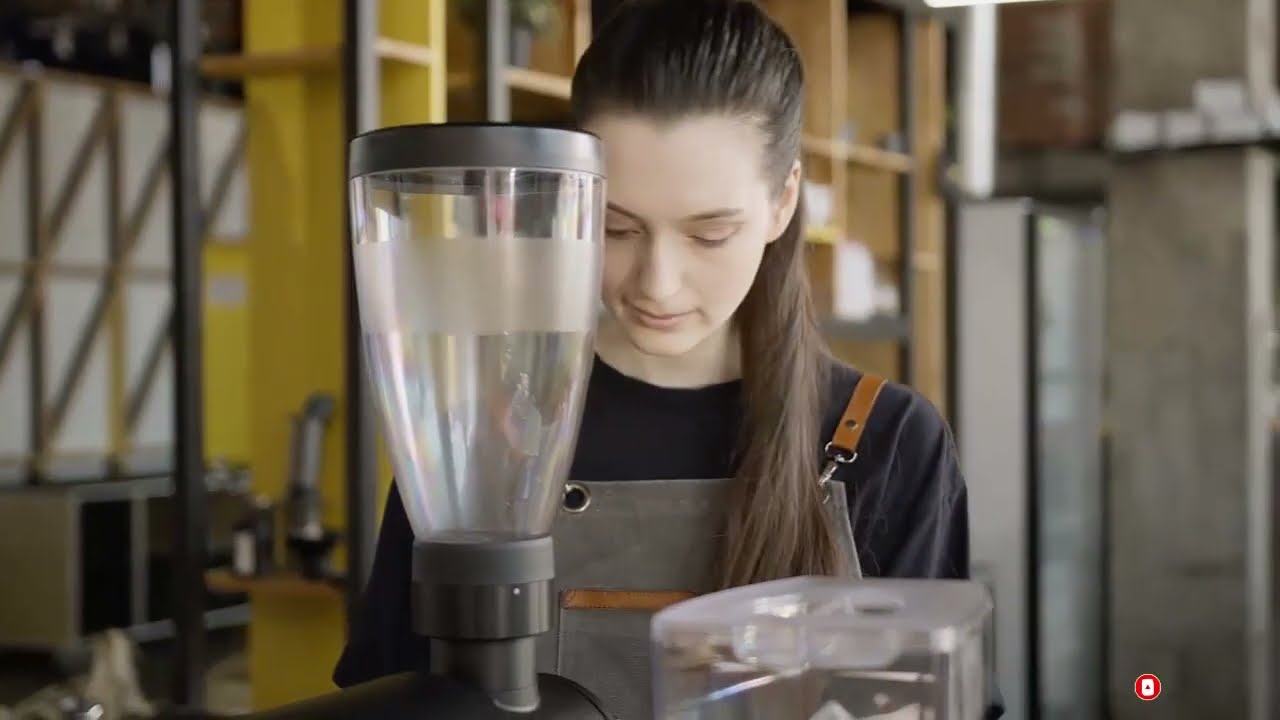In this construction or remodeling space, a young woman with long brown hair tied into a ponytail and some strands falling by her face, stands absorbed in her task. She wears a blue shirt under gray overalls with a brown strap. In front of her is a complex apparatus that resembles a blender attached to a large machine, featuring a transparent box which obscures its exact function. The background is a blurred mix of the unfinished building’s frame, with elements suggesting the spaces within it might be for a kitchen or a coffee shop. Notable details include a concrete pillar with some white at the top, several shelves (brown, yellow, and gray) holding various items including what looks like condiments and a possible salt shaker, and a gray wall with a cabinet below it featuring brown V-shaped slats. In the lower left corner, there seem to be pipes and what looks like an air conditioning unit. Shadows and structural features suggest a work in progress within this open framework environment.